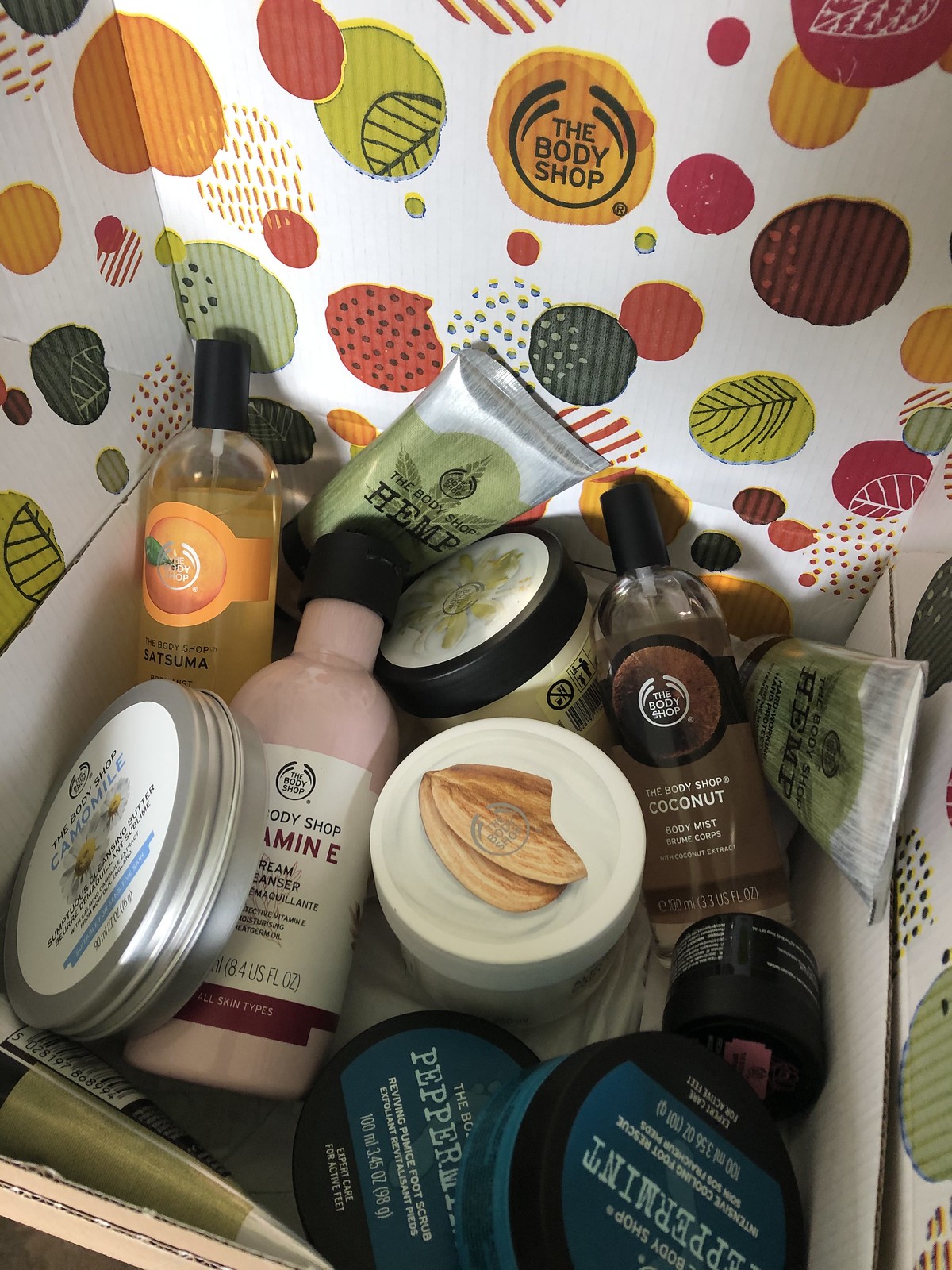This photograph captures a top-down view into a cardboard box filled with various skincare and body care products. The inside lid of the box features decorative brown patterns adorned with green, orange, and red accents, each containing small dots and stripes. Prominently displayed within these patterns is a branding element from The Body Shop, written in black ink on an orange background with black circles surrounding it.

Inside the box, several tins resembling shoe polish containers are visible. These tins are labeled with chamomile and peppermint marked in green. Also included is a pink bottle with a white label that reads "Body Shop Vitamin E." Additionally, there is a tube resembling toothpaste, characterized by its silver top and green body with a black label stating "hemp." On the right side, a clear bottle is present, bearing The Body Shop logo, and below it, the text "The Body Shop's Coconut Body Mist."